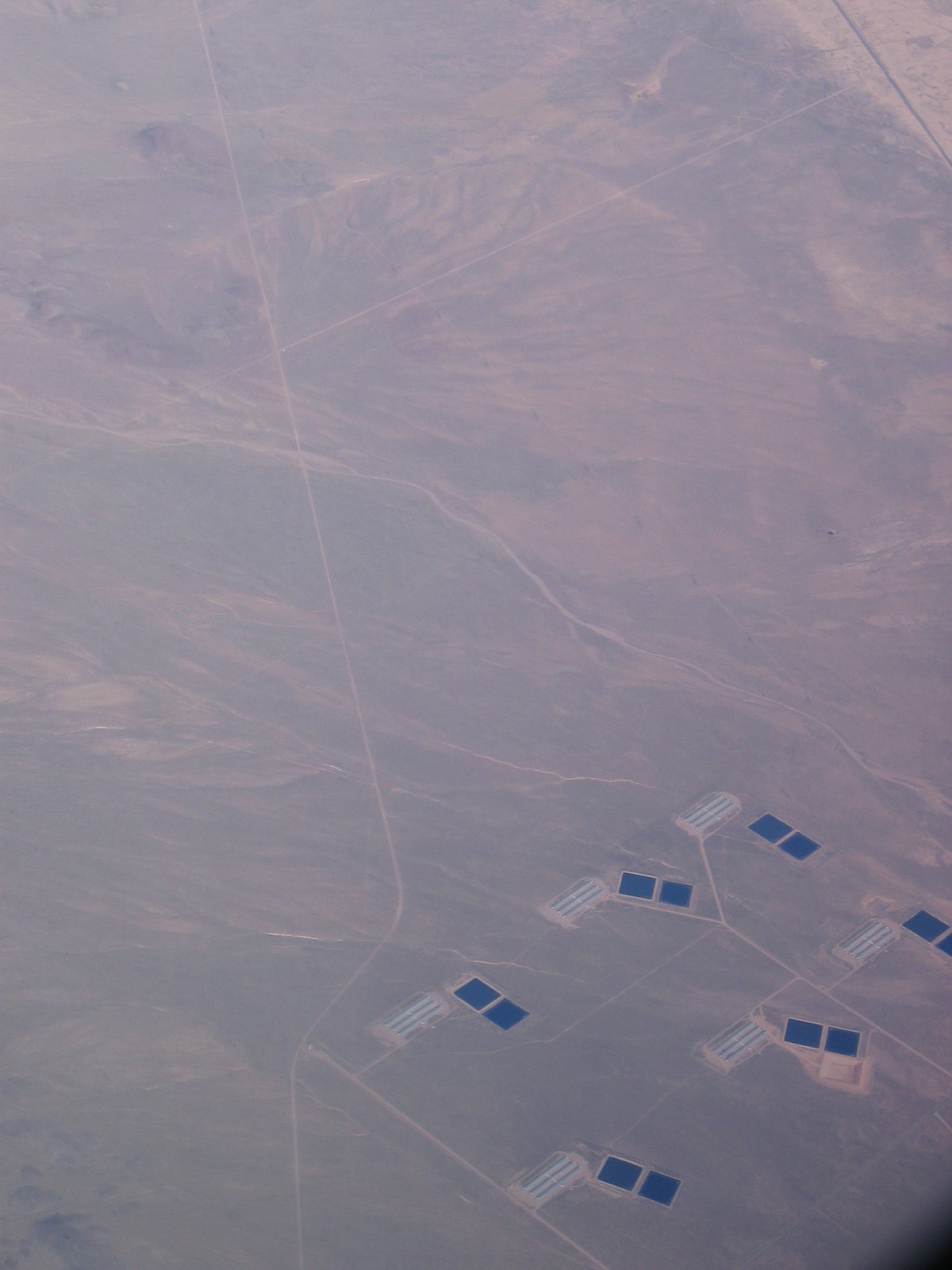This is a high-altitude aerial photograph, likely taken from a plane. It captures a vast, hilly landscape characterized by a pinkish-gray, brown mass of color. The terrain appears mountainous and barren, with sparse distinguishing features aside from the various roads that weave through the hills. In the bottom right corner of the image, there is a noticeable cluster of structures, possibly buildings, described by several small, light blue rectangles. Adjacent to these buildings are six pairs of darker square shapes, possibly swimming pools or solar panels. Additionally, one of these buildings has a distinct light brown area attached to it.